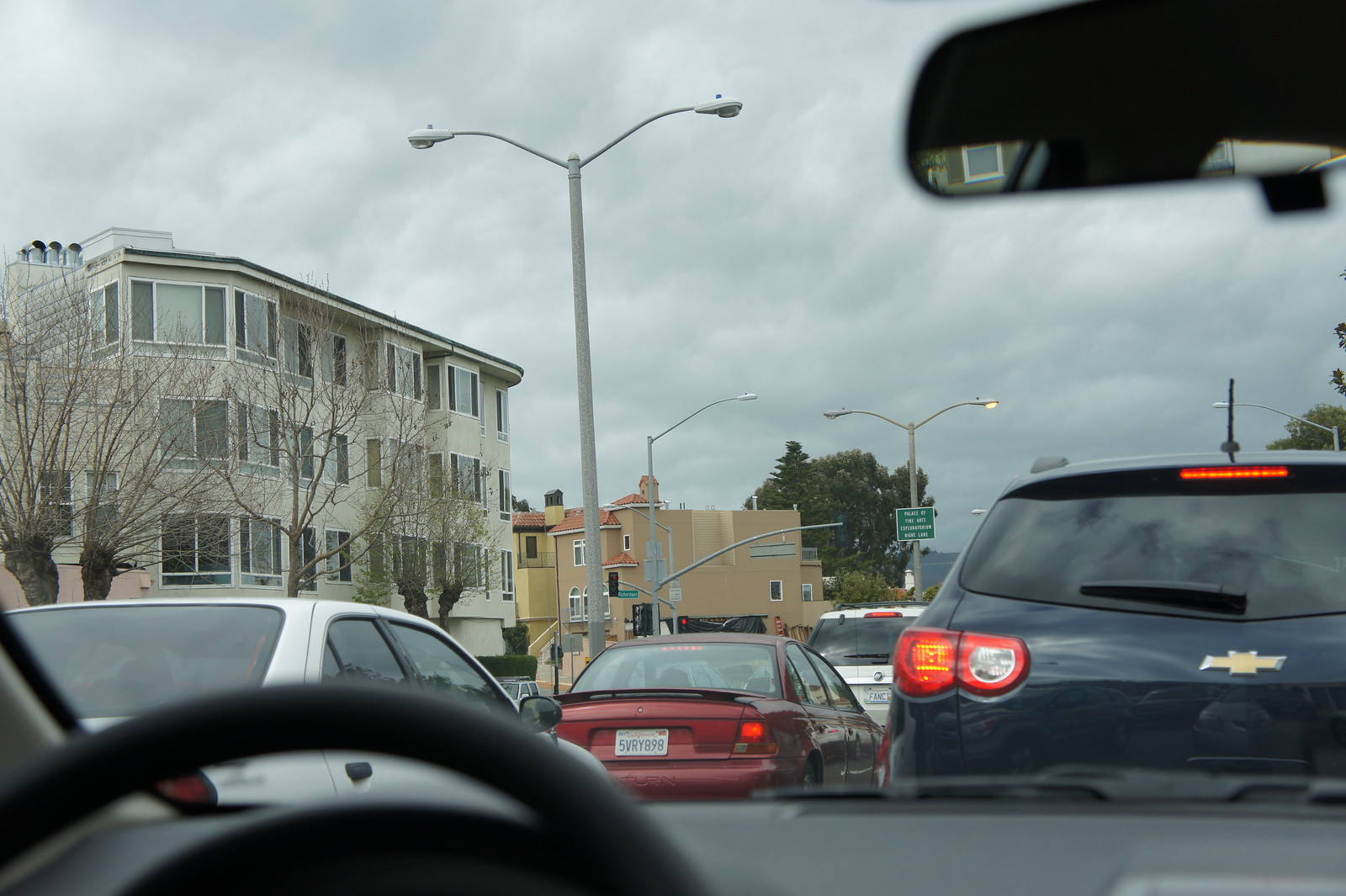This photograph, captured from inside a car with a view through the front windshield, depicts a scene of a traffic queue likely in an American city. The bottom part of the image features a slightly blurred black steering wheel and dashboard, indicating the photo is taken from the driver’s seat. Dominating the scene just ahead is a black Chevrolet SUV with its brake lights on. To the left, a line of parked cars includes a white sedan and a red car among others.

On the left side of the image, there are a few-story tall buildings, possibly apartments or hotels, with multiple windows. These buildings are fronted by a tree and accompanied by a row of light poles. The right side of the image reveals more trees and additional light poles in the distance. The sky overhead is entirely gray and cloud-filled, adding to the overall ambiance of a typical overcast day. This detailed portrayal captures the essence of waiting in traffic amidst urban surroundings.